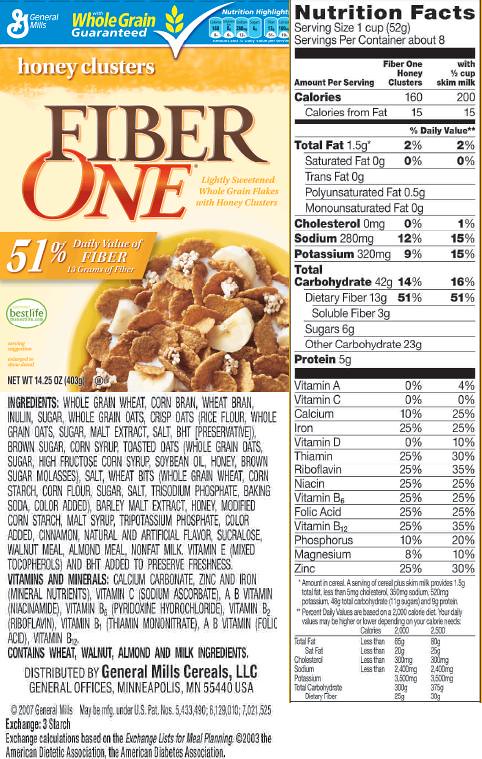This image is of a vertical rectangle that appears to be the back panel of a General Mills Fiber One cereal box. The background is predominantly white with black text detailing the nutritional information on the right side of the panel. At the top right, it reads "Nutrition Facts". The serving size is specified as 1 cup (52g), with about 8 servings per container. Following this, the nutritional breakdown includes calories, total fat, cholesterol, sodium, potassium, total carbohydrates, protein, and various vitamins.

On the left side of the panel, a section displays the front cover of the cereal box, possibly repeated on the back. At the top left corner, a blue banner features the "General Mills Whole Grain Guaranteed" logo, adorned with a white checkmark and a yellow grain symbol. Below this, a smaller yellow banner reads "Honey Clusters" in white text. The main beige section displays "Fiber" in brown font and "1" in red font, with another yellow banner noting "51% daily dose of fiber." An image of a bowl of the cereal, which is brown with what appears to be banana slices, is prominently shown. Beneath the bowl, black text lists the ingredients, vitamins, minerals, and other contents. The panel concludes with a note stating that the cereal is distributed by General Mills Cereals.